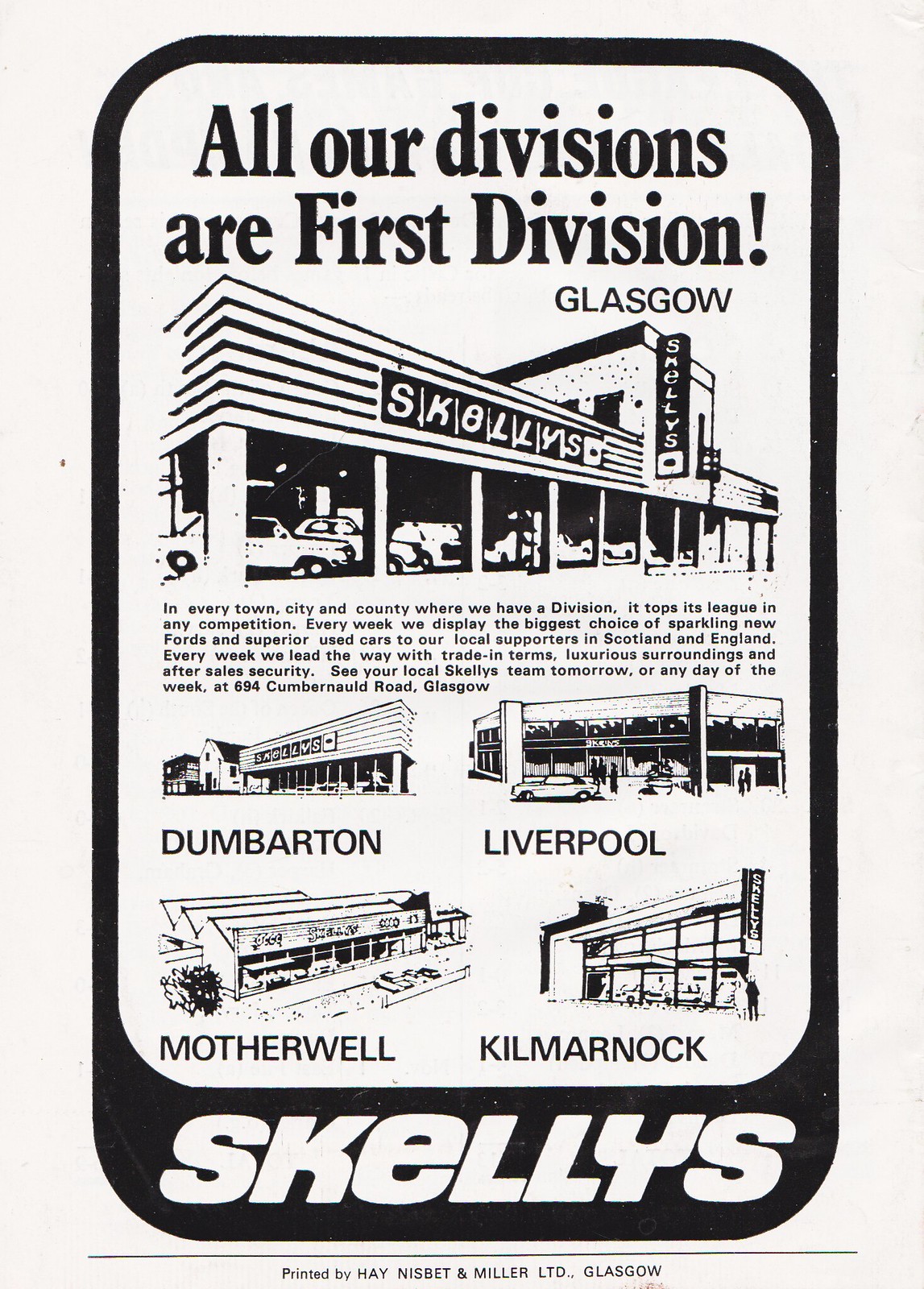The advertisement is a vintage black-and-white poster on aged white paper with a prominent black border at the bottom, which features the name "Skelly's" in bold, all-caps text. The ad is for Skelly's automotive company, highlighting their outstanding divisions across several cities. At the top, it states, "Our divisions, our first division, Glasgow," emphasizing their top positions in Glasgow and beyond. The ad details Skelly's locations in Dumbarton, Liverpool, Motherwell, and Kilmarnock, showcasing sketches of each building. The text mentions that Skelly's offers the widest range of new and superior used cars, ensuring luxurious surroundings, competitive trade-in terms, and dependable after-sales security. The central portion of the ad features black-and-white images of the cars and buildings related to each division, highlighting the extensive reach of Skelly's in both Scotland and England. The address for their Glasgow location is given as 694 Cumbernauld Road, urging local supporters to visit anytime to experience their leading automotive services.